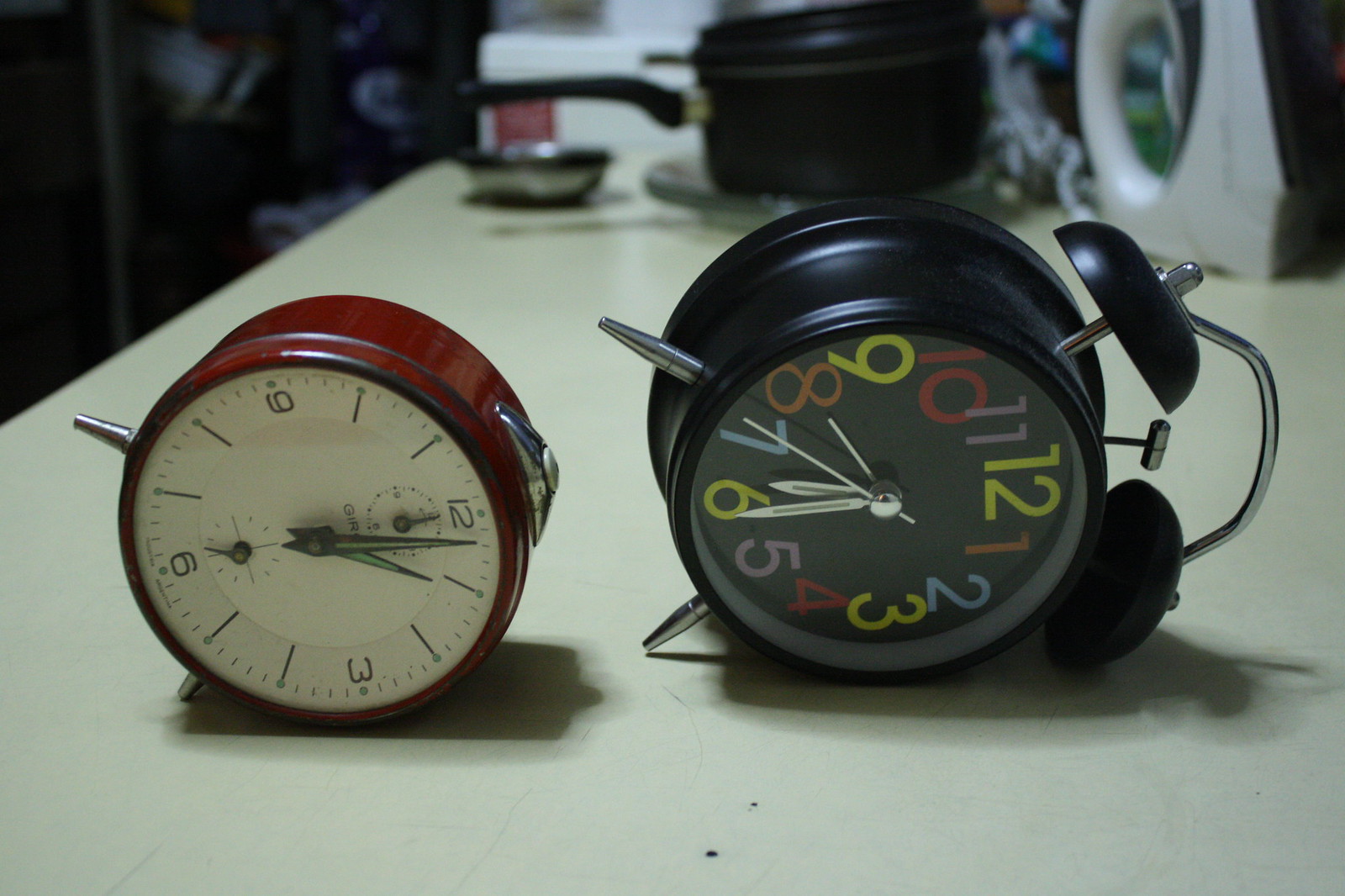The image displays two distinctive alarm clocks, juxtaposing styles from different eras. On the right side, there is a retro-themed alarm clock with a black casing. Its face is a vibrant mix of colors—yellow, pink, purple, red, orange, and blue—with artistically overlapping numbers, evoking a strong 1980s aesthetic. The clock is positioned on its side, upon an aged white table that has darkened over time. 

To the left, there is an older, more traditional alarm clock, characterized by its mahogany or dark wood exterior. Unlike the colorful clock, this one features a simpler design with only the cardinal numbers—3, 6, 9, and 12—indicated on its face. A small, secondary dial at the top of the clock displays the second hand, set against a yellowish-white background. The contrasting designs of the two clocks highlight the evolution of style and function in timekeeping devices.